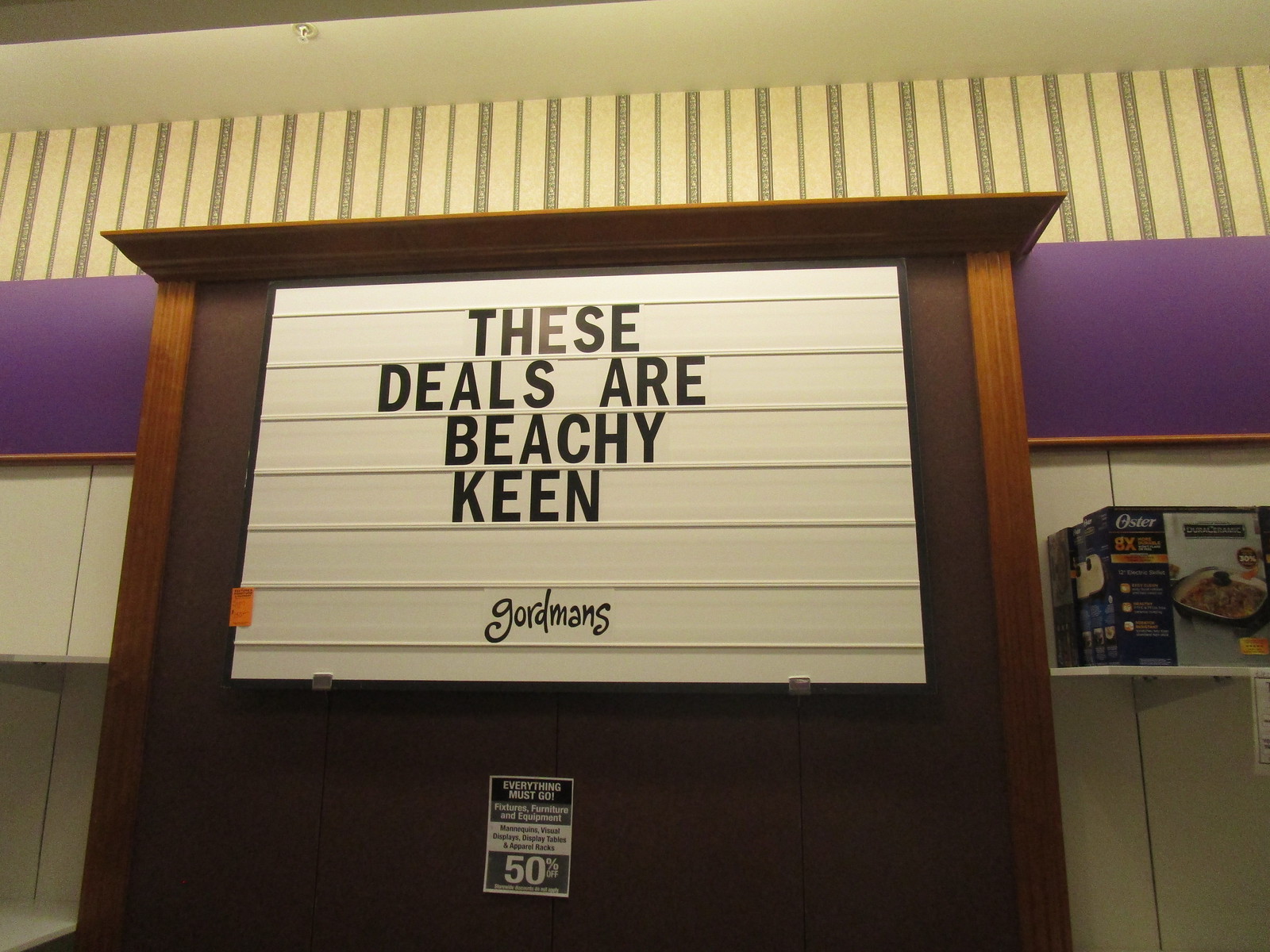In this indoor store display, a beige wall serves as the background, adorned with a horizontal purple line near the top. Below the line, shelves filled with various products, including boxes with the brand name Oster and what appears to be a casserole dish, suggest a kitchenware section. At the center of the display is a prominent wooden frame holding a rectangular white sign with black lettering. The sign declares, “These deals are B.C. King's, Goldman's” or “Beaky Keene, Gordman's” amid some confusion over the exact wording. Attached below the main sign is a black and white tag stating “50% off,” hinting at significant discounts. The backdrop of the display incorporates brown vertical lines and a purple fixture, possibly remnants from the store’s previous layout. Overall, the store seems to be undergoing a liquidation sale, as indicated by phrases like “everything must go” and “fixtures, furniture, and equipment, 50% off," suggesting it might be closing down.